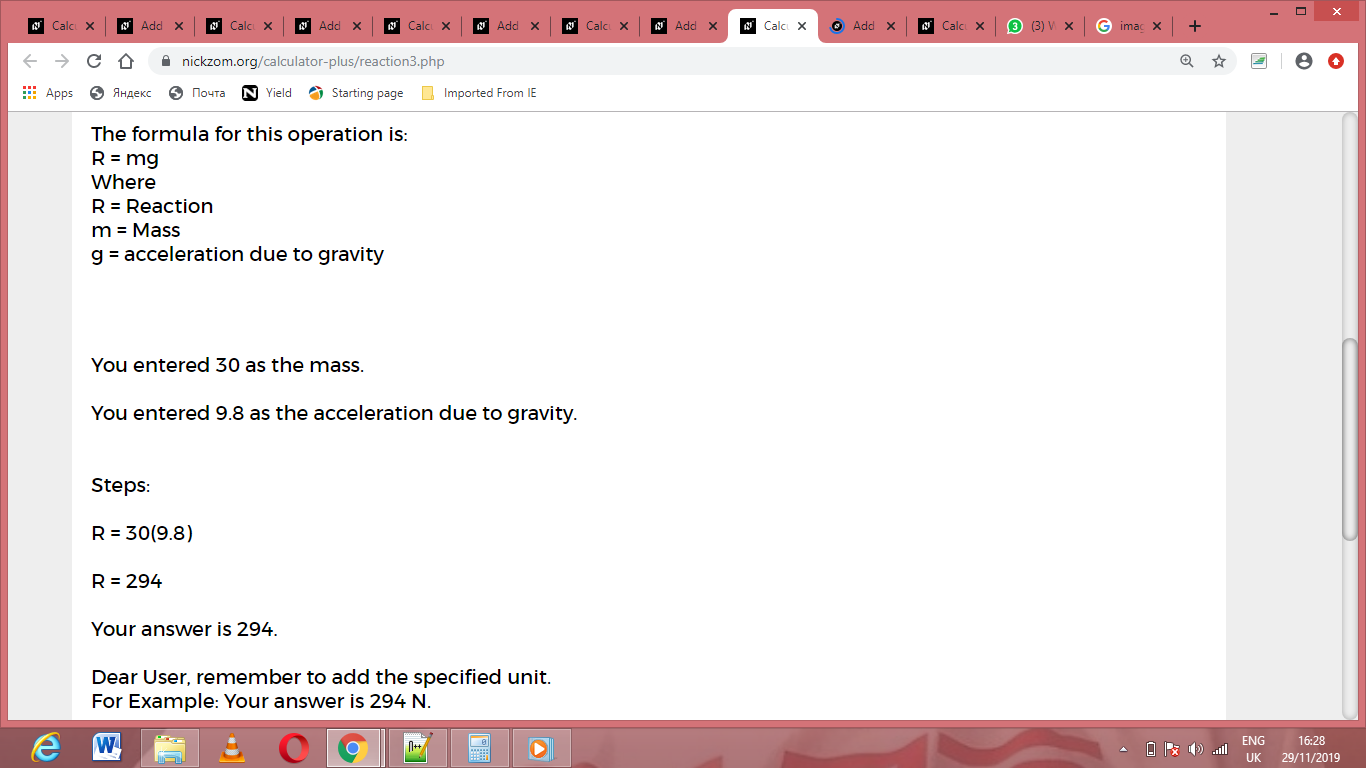**Description:**

The image is a screenshot of an individual's desktop, characterized by a rose-colored theme that serves as the background for all the icons and tabs displayed. The desktop is notably cluttered, with 14 open tabs, 9 of which belong to the same website, www.nickzum.org. Among these tabs, an additional one is open, suggesting continuous engagement with this site. Other notable tabs include a blue icon, indicating either a separate webpage or application, a Skype or WhatsApp call in progress, and a Google search page.

In the browser interface, familiar navigation tools such as the left and right arrows, refresh button, home button, and the address bar with a lock symbol (revealing the secure connection to nickzum.org) are visible. The specific page displayed is 'calculatorplusreaction3.php', presenting a text document that delineates a physics formula for calculating reaction force, specified as \( r = mg \). The sample calculation entered shows:
- Mass (\( m \)) = 30 kg
- Acceleration due to gravity (\( g \)) = 9.8 m/s²
- Resulting reaction force (\( r \)) = 294 N, annotated with a reminder for the user to include the unit 'N' (Newton).

The desktop also features a variety of application icons strewn across the screen. Notable icons include:
- Internet Explorer logo
- Microsoft Word file logo
- VLC media player's traffic cone logo
- Opera browser icon
- Google Chrome icon
- Windows Media Player icon
- Notepad application
- An unrecognizable icon, suggesting either a non-standard or obscure application.

The combined elements of the rose-themed desktop, and numerous open tabs and applications signify an individual deeply engrossed in multi-tasking activities, possibly balancing communication, research, and media consumption.